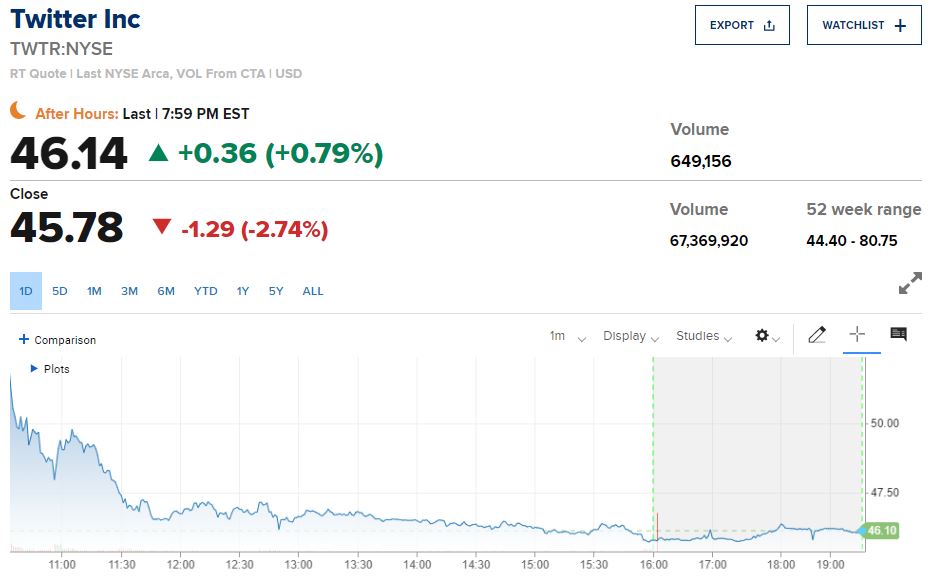The image displays financial information for Twitter Inc. (NYSE: TWTR) on a white background. Key details include:

- **Real-Time Quotes:** Featuring data from NYSE ARCA and CTAUSD with options for Export and adding to a Watchlist.
- **After Hours Trading:** Showing the last recorded value at 7:59 p.m. EST, with the stock priced at $46.14, up $0.36 (+0.79%) indicated by a green arrow.
- **Day Close:** With a closing price of $45.78, down $1.29 (-2.74%) as shown by a red arrow.
- **Volume:** Reporting a regular volume of 67,369,920 and an after-hours volume of 649,156.
- **52-Week Range:** Spanning from $44.40 to $80.75.
- **Time Frames:** Navigation options for different time frames, including 1D (highlighted in blue), 5D, 1M, 3M, 6M, YTD, 1Y, 5Y, and All.
- **Chart:** At the bottom, depicting price movements with markers at intervals such as 11, 11.3, 12, 12.3, and 13.